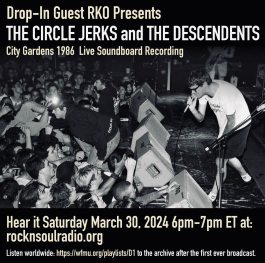This is a black-and-white poster advertisement for a music event featuring an album cover or a live soundboard recording with the prominent title "RKO Presents the Circle Jerks and the Descendants." The event, labeled as “City Gardens 1986 Live Soundboard Recording,” is centralized at the top of the poster. Beneath the text, there's a striking photograph capturing the energetic performance of the Circle Jerks. The lead vocalist is depicted in a white shirt, sunglasses, black shorts, white socks, and black shoes, passionately singing into a microphone towards an enthusiastic crowd. The stage is illuminated with box-like gray lights, and additional microphone stands are visible. The audience, composed mostly of young men, is seen cheering and some are crowd surfing. Below the image, it reads: "Hear it Saturday, March 30th, 2024, 6-7 p.m. Eastern Time at rockandsoulradio.org." Additional smaller text underneath, though partly illegible, suggests that the broadcast can be accessed worldwide through a specified archive link. The entire composition of the poster conveys the raw and electrifying essence of a live punk rock concert.